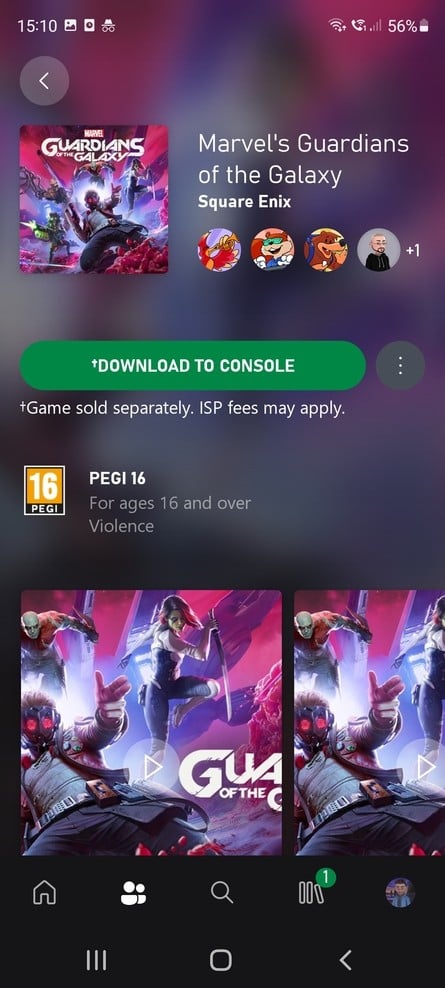The image is a screenshot taken from a mobile phone at 15:10, indicated at the top left corner along with three small icons: one for an image, one possibly for voice recording, and another indistinguishable small icon. On the top right are typical phone status icons, all in white, showing battery life, signal strength, Wi-Fi connectivity, and a telephone call icon.

Just below this, to the left, there's a white arrow pointing left within a gray circle. Beneath that is artwork from the video game "Guardians of the Galaxy." The artwork features the title "Guardians of the Galaxy" in white text and depicts the character Star-Lord sliding forward with his fingers mimicking guns. Other Guardians of the Galaxy characters are seen in the background, set against a red-purplish hue.

To the center and right of the image, the text "Guardians of the Galaxy, Square Enix" appears in white, alongside four circular avatars representing other players currently involved in the game. Below this, there's a green rectangular button with rounded edges that reads "Download to Console" in white. Next to it, within a larger gray circle, are three vertical dots.

Further down, the text "Games sold separately, ISP fees may apply" is displayed in white. There's also a PEGI 16 rating logo—a yellow square with a white border—labeling the game as suitable for ages 16 and over due to violence.

Near the bottom, the same artwork is repeated, showing Star-Lord with finger guns and the other Guardians in the background. Beneath this, a set of icons is lined up: a home button, a two-silhouette icon, a magnifying glass, a three-book icon with the right book slightly tilted bearing a green circle with the number one, and a small avatar of an indistinguishable white man.

At the very bottom, additional mobile navigation buttons appear: a back button, a home button, and three horizontal lines. The general background of the image is a light gray with purple, which appears to be a blurred representation of the artwork for "Guardians of the Galaxy."